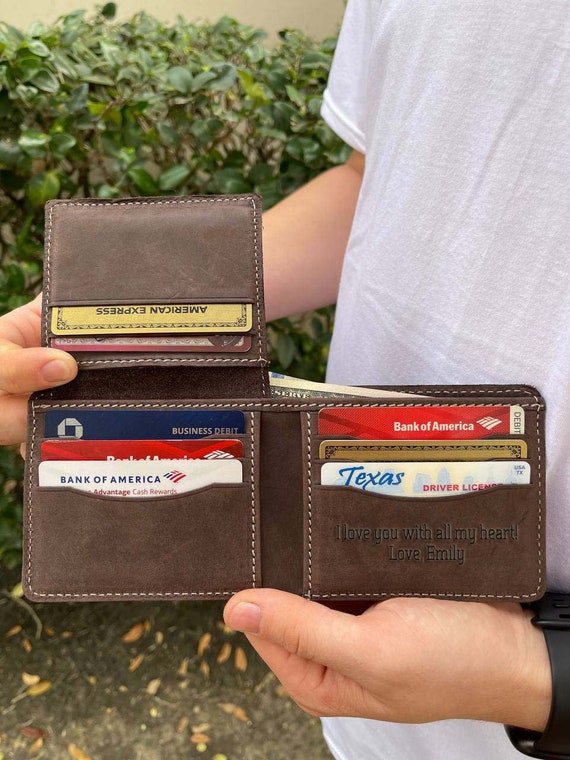The image is a full-color, horizontally-oriented photograph of a white person holding an open brown leather wallet with white stitching, taken outdoors against a background of a shrub and some grass. The person, wearing a white short-sleeved shirt and a black wristwatch, displays the wallet prominently in the foreground. The wallet features an engraving that reads, "I love you with all my heart. Love, Emily." Inside, the wallet's three fold-out pockets reveal a Texas driver's license, two Bank of America cards (one white and one red), an American Express card, a Chase card, and another business debit card. Additionally, some American currency is partially visible, peeking out from the money storage area. The photo appears to focus on the details and contents of the wallet, likely as a product shot to showcase its various compartments and personal touches.